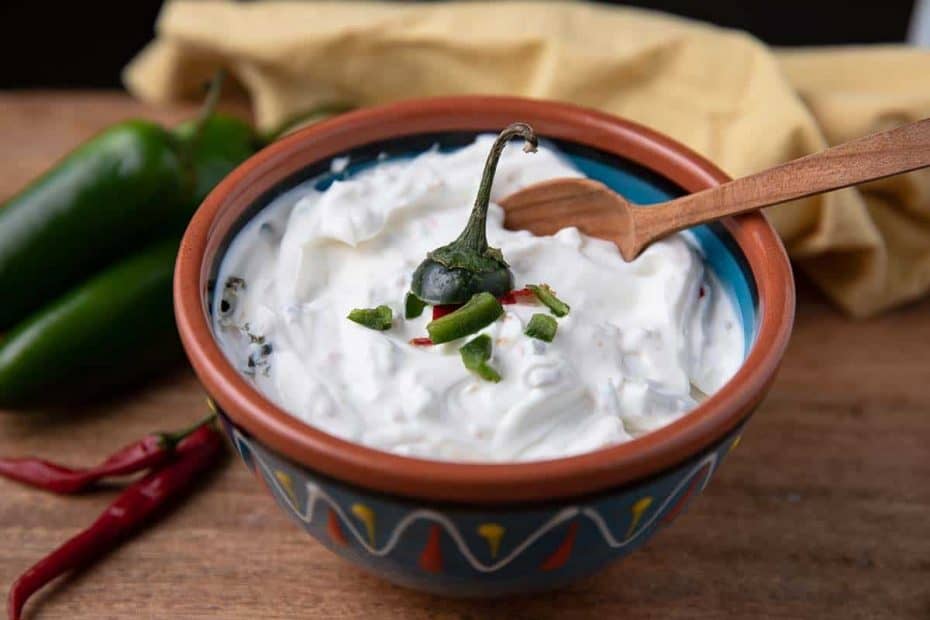This photographic image captures a bowl that appears to be made of china with intricate, colorful designs. The bowl itself has a brown rim and a blue body adorned with yellow squiggles and red and yellow decorative elements. It is filled with what looks like chunky sour cream or a creamy dip, accented by a green pepper protruding from the center and garnished with chopped pieces of scallion. A wooden spoon rests on the right side of the bowl. The bowl is placed on a brown wooden table, and in the background, slightly out of focus, are two red chili peppers and two green peppers positioned to the left. Behind the bowl, there is a crumpled brown cloth or towel, adding a rustic element to the scene. The photo is taken from a slightly angled, top-down perspective, in an indoor setting with no text present in the image.